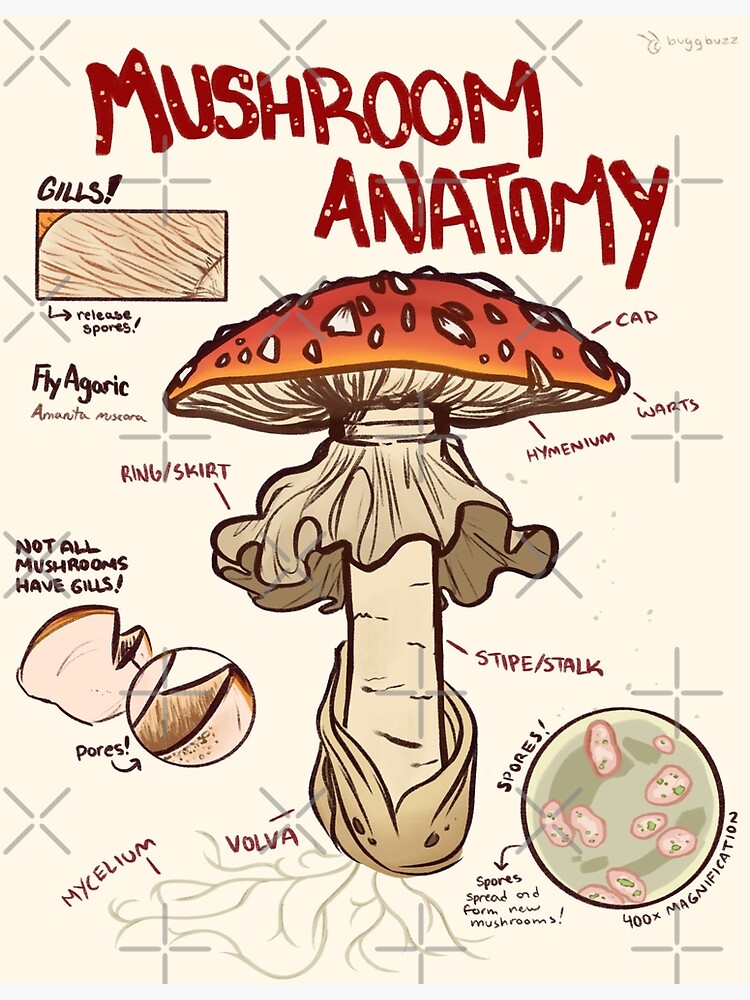The image is a detailed, vertically oriented diagram of mushroom anatomy, crafted in a cartoon style, set against a white background. At the top center, in large red font with white speckles, it reads "Mushroom Anatomy." The focal point is a large sketch of an orange-topped mushroom featuring a grey stem, labeled meticulously with various parts. The cap is pointed out with an arrow, indicating white patches called warts. The underside of the cap, labeled hymenium, shows gills above a smaller rectangular close-up. A frilly structure at the top of the stem, labeled ring/skirt, is depicted along with the stipe/stalk of the mushroom.

An accompanying close-up box displays additional details such as the gills, which release spores. Beneath this, it notes "Fly Agaric, Amanita muscaria." Near the bottom of the main mushroom sketch, text indicates "Not all mushrooms have gills," pointing to a part labeled pores. To the right, a circular inset shows spores at 400X magnification with a note: "Spores spread and form new mushrooms."

In the upper right corner is a faint logo appearing to spell "BUGBUZZ," with a watermark visible throughout the image at various angles. Another frilly structure at the stem's bottom, labeled vulva, is also indicated. The diagram is comprehensive, with a clear emphasis on both the shared and unique features of the mushroom anatomy.